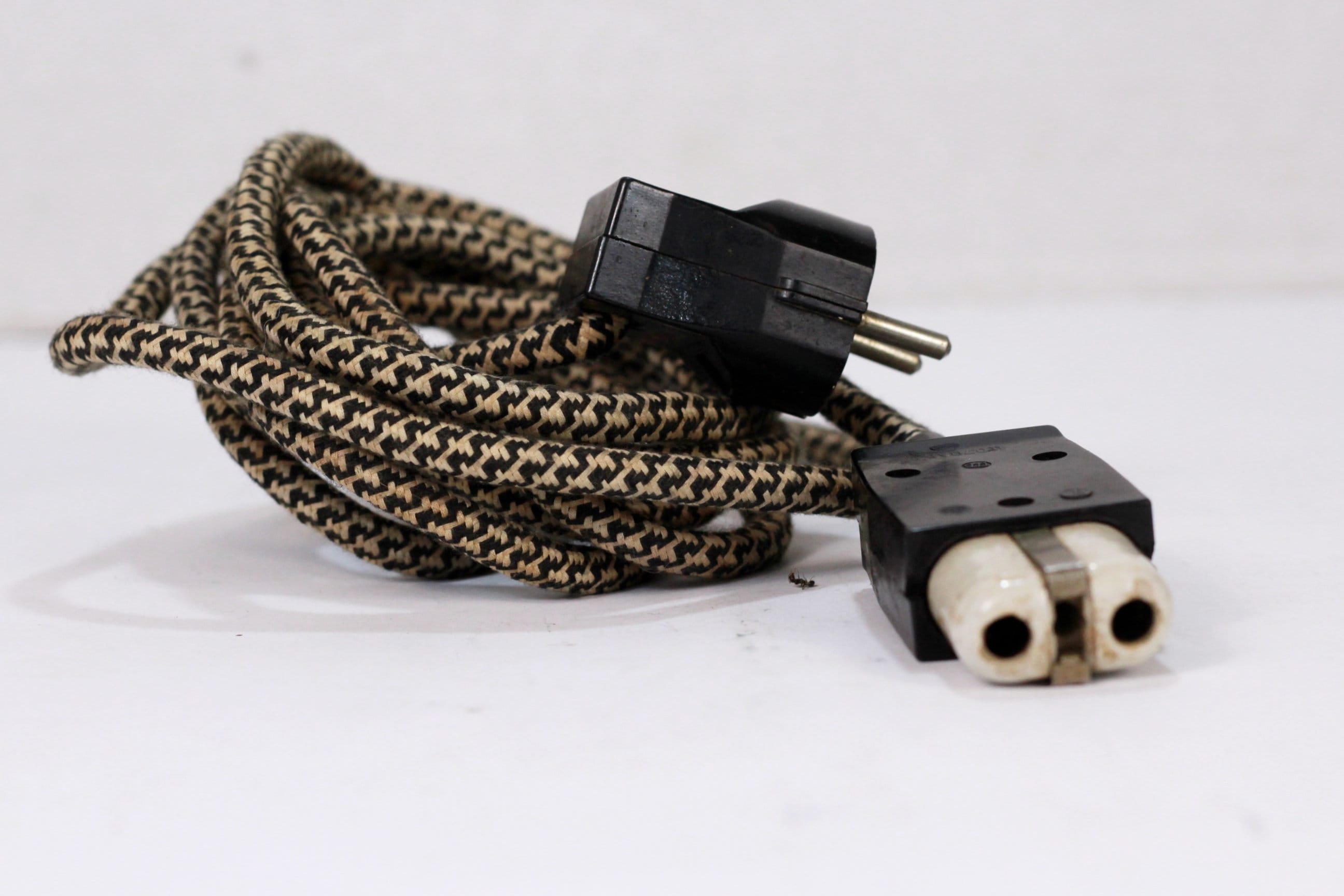This is a close-up photograph of an old-fashioned extension cord against a white background, which could be a white table or floor, blending into a white wall. The cord itself features a thick, woven cloth sheath in beige and brown with a zigzag pattern, giving it a vintage feel reminiscent of the 1950s. The cable is coiled into a neat loop, resembling a snake. One end of the cord has a dark brown plastic casing with two gold prongs, indicating the plug, while the other end features a slightly burned or dirty dark brown plastic receptacle with two white, cylindrical holes that contain silver inserts, likely designed for plugging in devices. The absence of a ground connector on either side further suggests its age and possibly foreign origin. Additionally, a small crumb or dead ant is visible next to the coiled cable.